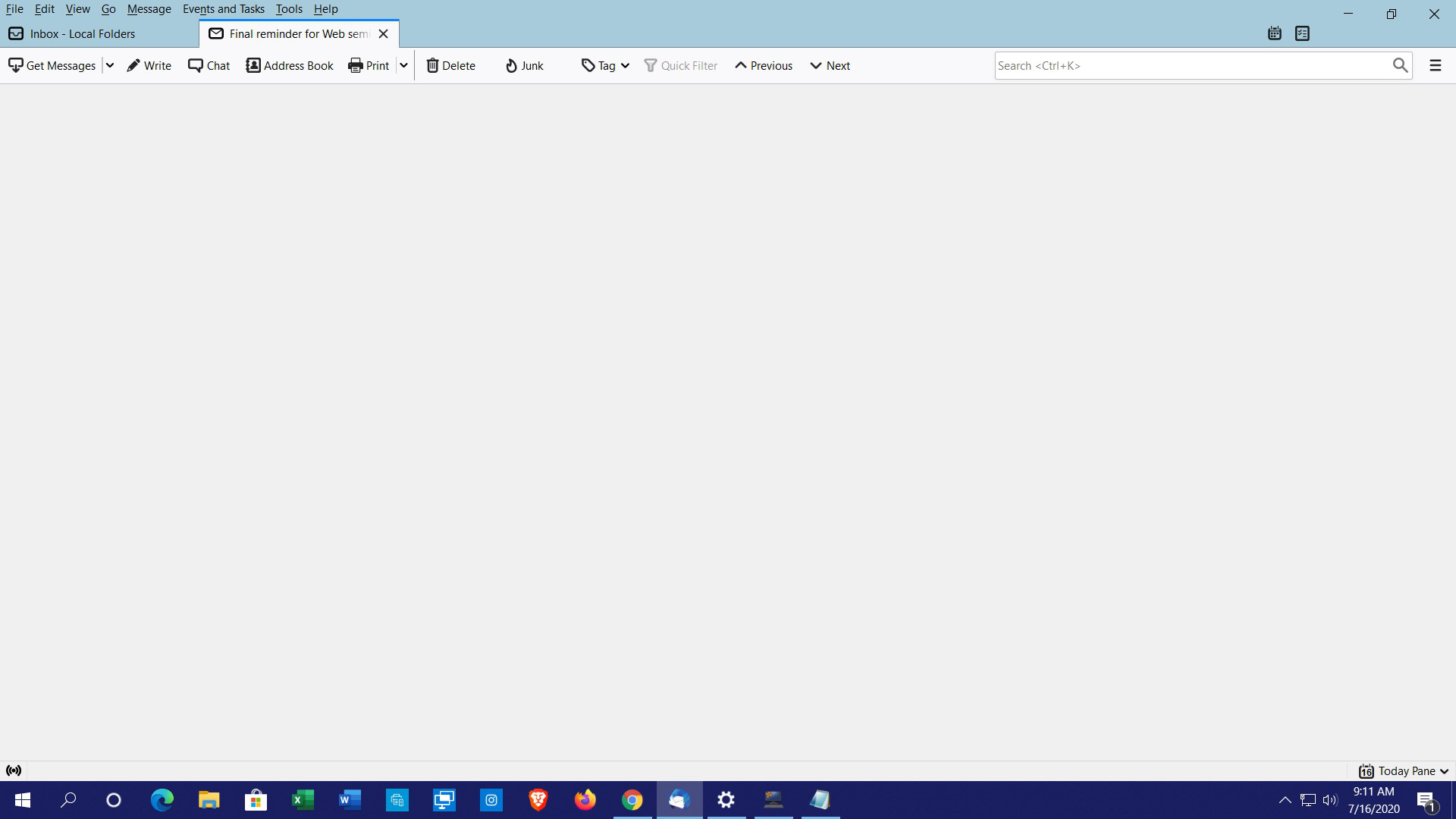The image depicts a screenshot of an email client program with a typical user interface layout. At the top-left corner, there is a menu bar displaying options such as "File," "Edit," "View," "Go," "Message," "Events and Tasks," "Tools," and "Help." Below this, there's a navigation pane with "Inbox" and "Local Folders" labels, and an additional tab labeled "Final Reminder for Web," though the last word is partially cut off. 

Immediately beneath this, there is a toolbar with buttons for "Get Messages," "Write," "Chat," "Address Book," "Print," "Delete," "Junk," "Tag," "Quick Filter," "Previous," "Next," and on the far right, a search bar. 

The main section of the screenshot displays a plain gray-black background with no visible messages or content. 

At the bottom of the screen, the Windows taskbar is visible. It includes the Windows icon, a search bar, shortcuts to Microsoft Edge, File Explorer, Microsoft Store, Google Chrome, settings, and other applications. On the bottom right corner, the date and time are displayed as 9:11 AM on July 16, 2020.